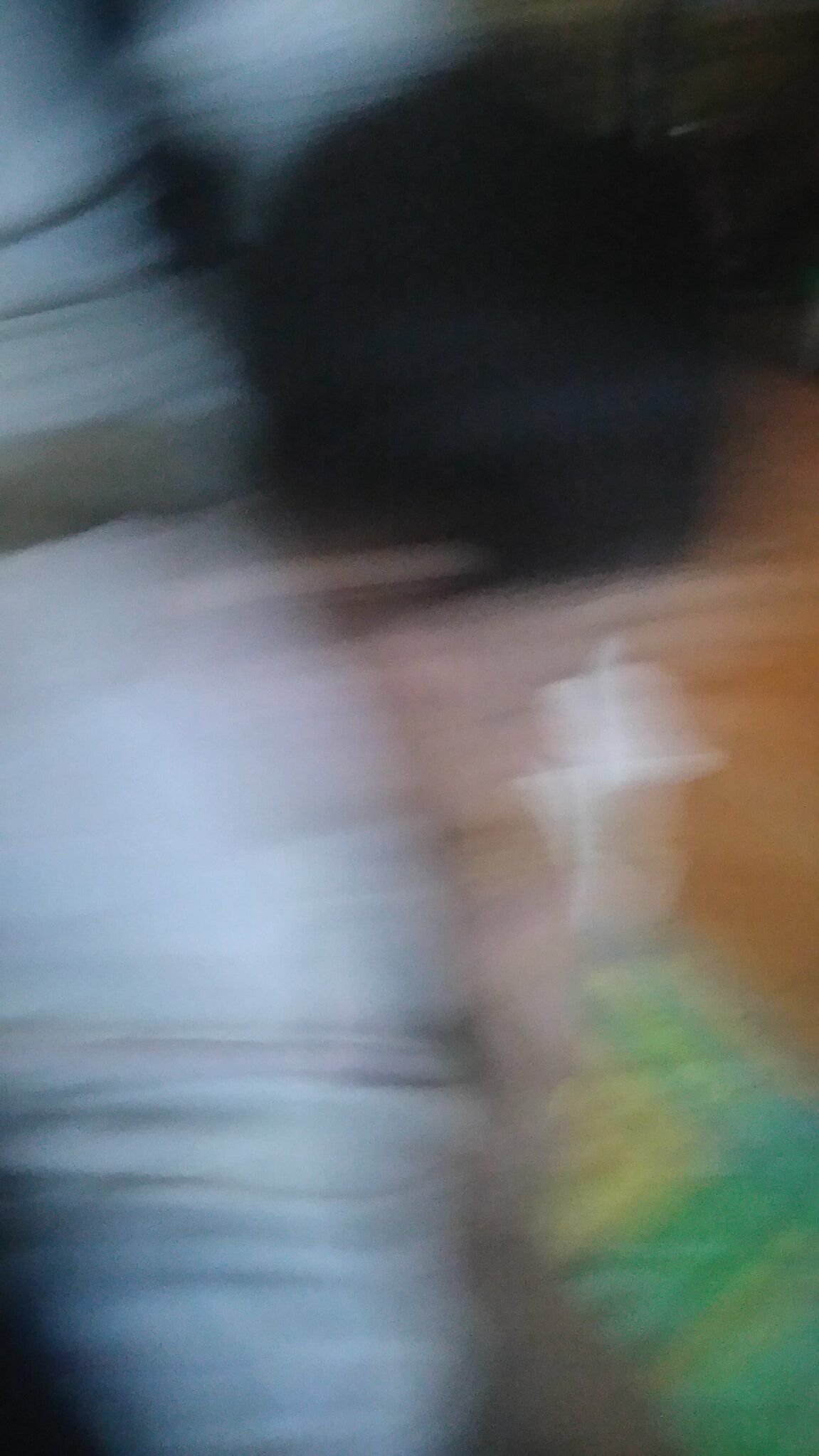This extremely blurred and out-of-focus color photograph captures an unclear, dynamic scene that implies the camera was rapidly moved during the shot, resulting in significant motion blur. Towards the top of the image, a dark area can be seen, possibly representing black hair or a shadowy region. Below this, on the upper left, there's a grey zone with horizontal black lines, possibly resembling a pillow or bedspread. The middle and lower sections feature a gradient from grey to blue-grey, with a small blue rectangle that vaguely suggests the leg of a person or denim jeans. 

On the right side of the image, there's a brown or tan area, potentially flesh-colored, but lacking clear outlines to identify a person. Adjacent to this brown section is a white figure that could be a cup with a protruding straw. Below this area, some green, yellow, and blue checkered fabric is discernible, possibly indicating rapid motion in this fabric pattern.

Overall, the photo lacks textual elements and seems to be captured indoors. All these blurred fragments and overlapping colors indicate a fast movement, creating an abstract and somewhat chaotic composition.